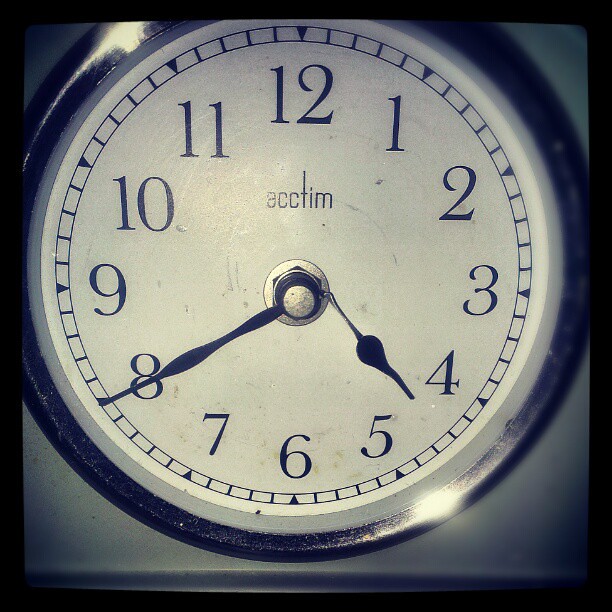This is a color photograph of a vintage-style clock with a round, silver outer casing. The clock's face is stark white, featuring crisp, black numerals that stand out clearly against the background. The black hands of the clock are positioned at approximately 4:40. Below the numeral 12, the brand name "ACCTIM" is prominently displayed in lowercase letters. The clock is set against a simple, gray backdrop, which contrasts with the clock's metallic sheen and clean design. The image is devoid of any additional elements such as people, animals, plants, buildings, or vehicles, allowing the viewer's focus to remain solely on the clock itself.